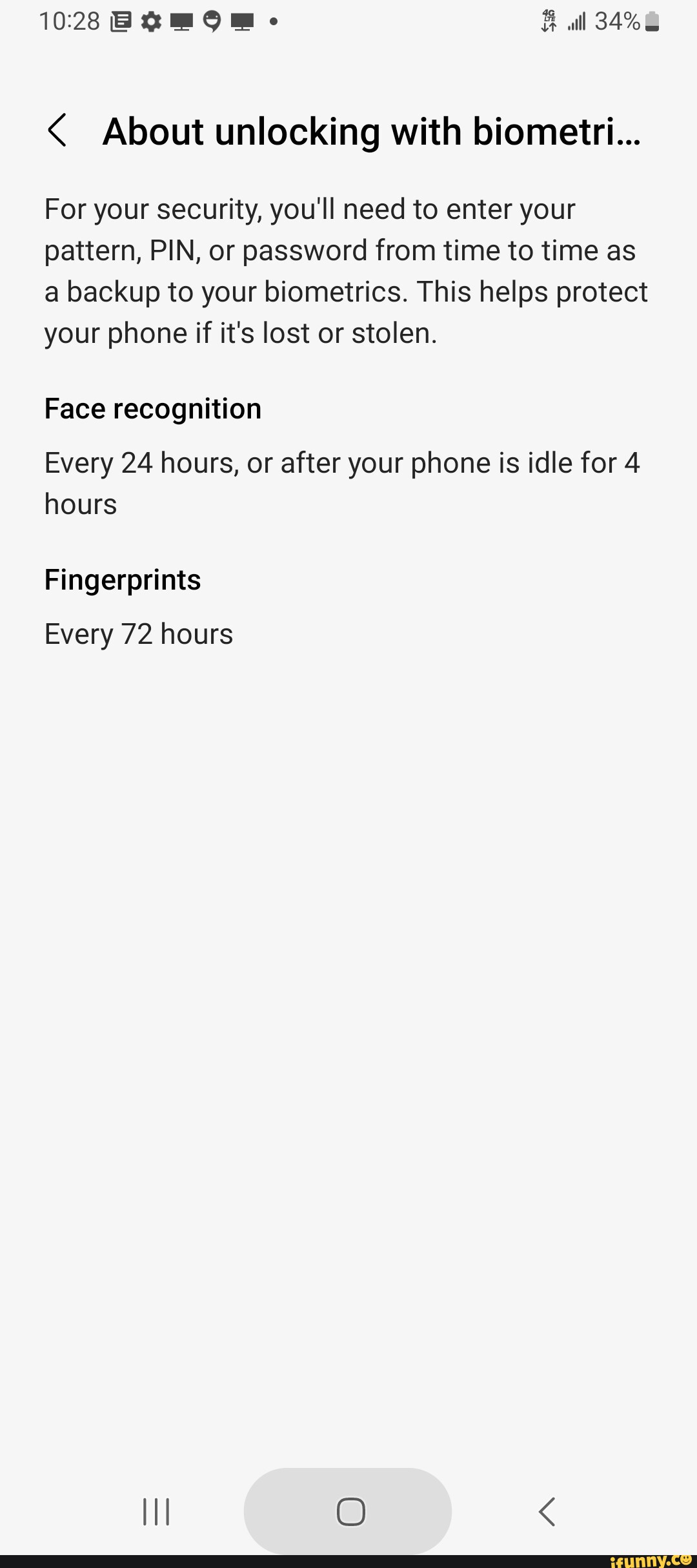In the screenshot captured on an Android device, the time displayed on the phone is 10:28, although it is unclear whether it is AM or PM. The phone's battery is at 34%, and there are a couple of notifications visible at the top. The focal point of the screenshot is a message discussing the use of biometrics for phone security. The message reads: "For your security, you'll need to enter your pattern, PIN, or password from time to time as a backup to your biometrics. This helps protect your phone if it's lost or stolen. Face recognition every 24 hours or after your phone is idle for four hours. Fingerprint is every 72 hours."

This security prompt is specific to Android devices, as indicated by the context and user familiarity with iPhone biometric systems, which differ in their configuration and settings. The message emphasizes the importance of regular security checks to ensure the device remains protected in case it is lost or stolen. Users can rely on biometrics such as facial recognition or fingerprint scans for quick access, but periodic input of a pattern, PIN, or password enhances security. This measure ensures that no one can duplicate a user's fingerprint or face, adding an extra layer of protection for those who prioritize the security of their personal information.